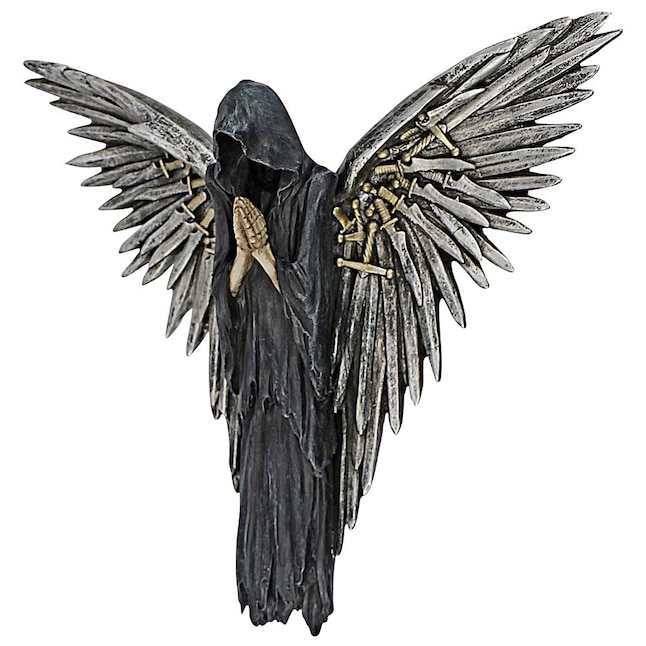A photorealistic image depicts a mysterious and eerie figure, likely representing the Angel of Death. The figure is cloaked in a long black, tattered robe with a hood that obscures its face, leaving nothing but an inky void where facial features would normally be. The figure is in a prayer-like stance, with skeletal hands emerging from the sleeves. Attached to the figure's back are two imposing wings constructed from numerous swords and knives of varying sizes. The swords have silver blades and gold handles, which are positioned towards the inner part of the wings, fanning outwards to form a menacing, spiked formation that looks like feathers. The scene is set against a stark white background, enhancing the dark and ominous presence of the angelic reaper. There are also hints of possible Japanese or Korean writing, though it's not clearly legible. The overall palette is dominated by black, with accents of gray, silver, and gold, creating a hauntingly captivating image.